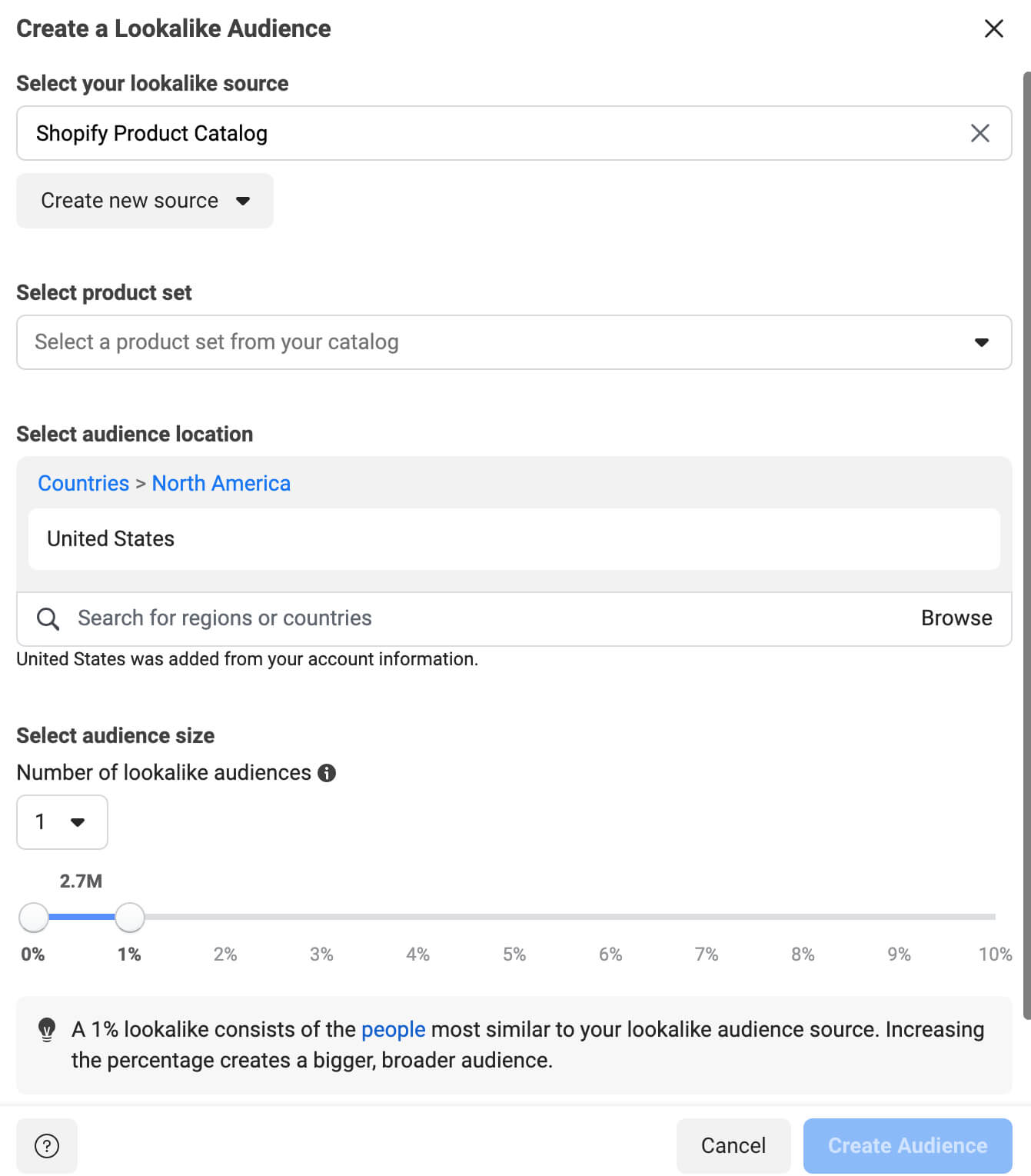The image shows a screenshot of a device displaying a user interface for creating a lookalike audience. The background color is white. In the top left corner, text reads, "Create a Lookalike Audience," while in the top right corner, there is a black "X" icon. Below this, the text "Select your Lookalike Source" is visible on the left side. Directly underneath, it reads "Shopify" (spelled S-H-O-P-I-F-Y) followed by "Product Category." 

Further down, there is a tab labeled "Create New Source." Below it, the text "Select Product Set" appears, followed by "Select a Product Set from Your Catalog." Continuing down, the text reads, "Select Audience Location." 

Under this section, the text "Countries" appears with a right-facing arrow next to it indicating North America, followed by "United States." 

In the following section, there is a magnifying glass icon next to the text "Search for Regions or Countries." To the far right of this section, the word "Browse" is visible. Finally, the text "United States was added" appears at the bottom.